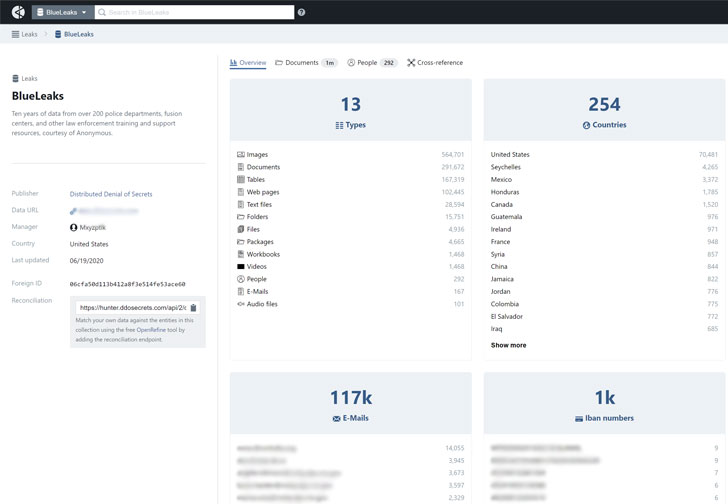At the top of the page, there is a black background with a somewhat blurry, rectangular-shaped section. On the left side of this section, there is a gray area with white text that seemingly reads "Blue Leaks." To the right of it, within a white area, there's a gray magnifying glass icon next to text that might say "search in" or "search on Blue Leaks." Adjacent to this is a gray circle containing a black question mark.

A gray border runs along the left-hand side of the page, featuring four gray lines and the word "Leaks." An arrow pointing to the right includes the text "Blue Leaks" in blue.

As the background transitions to white, the left-hand side displays the following text: "Leaks, Blue Leaks, 10 years of data from over 200 police departments, fusion centers, and other law enforcement training, support resources, courtesy of Anonymous." Below this description is a thin gray line, followed by more text that reads "Published" or "Distributed." 

Further down, text appears to mention "Now the secrets," though the data URL is blurred out. There is some information starting with "Manager, PXE" which is difficult to read, and text that states "Country: United States." The document notes the last update as "06/19/2020" and mentions "Foreign ID," but this information is partially obscured.

Lastly, a gray box on the side lists details such as "13 types," "254 countries," "117K emails," and "1K IBN numbers."